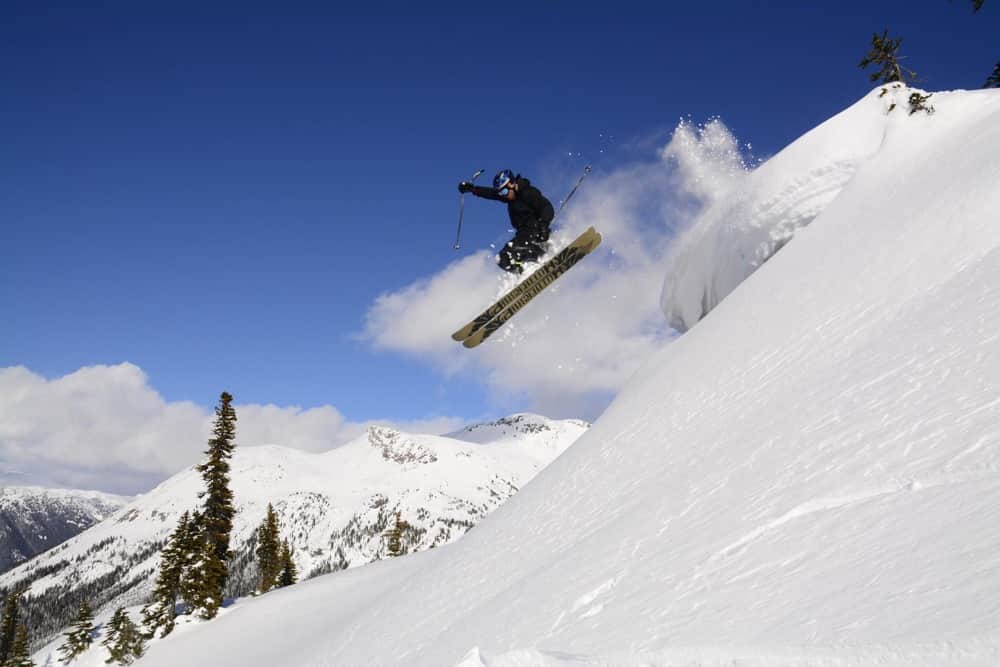In this dynamic outdoor landscape image, we see a skier, clad in a black jacket, black pants, and a helmet, performing a jump off a steep snow-covered hill. The skier, captured mid-air with snow flying off their yellow and black skis, holds ski poles in each hand, indicating the intensity of the moment. The bottom of the skis has some writing, though it's not legible. Dominating the right side of the image is the imposing snowbank the skier leaped from, while the left side reveals distant snowy mountains interspersed with tall green trees. Above these mountains, a puffy white cloud is visible, set against a backdrop of clear blue skies, which occupy much of the upper part of the photograph. The scene is serene with no signs of wind or snowfall, emphasizing the crisp winter day.